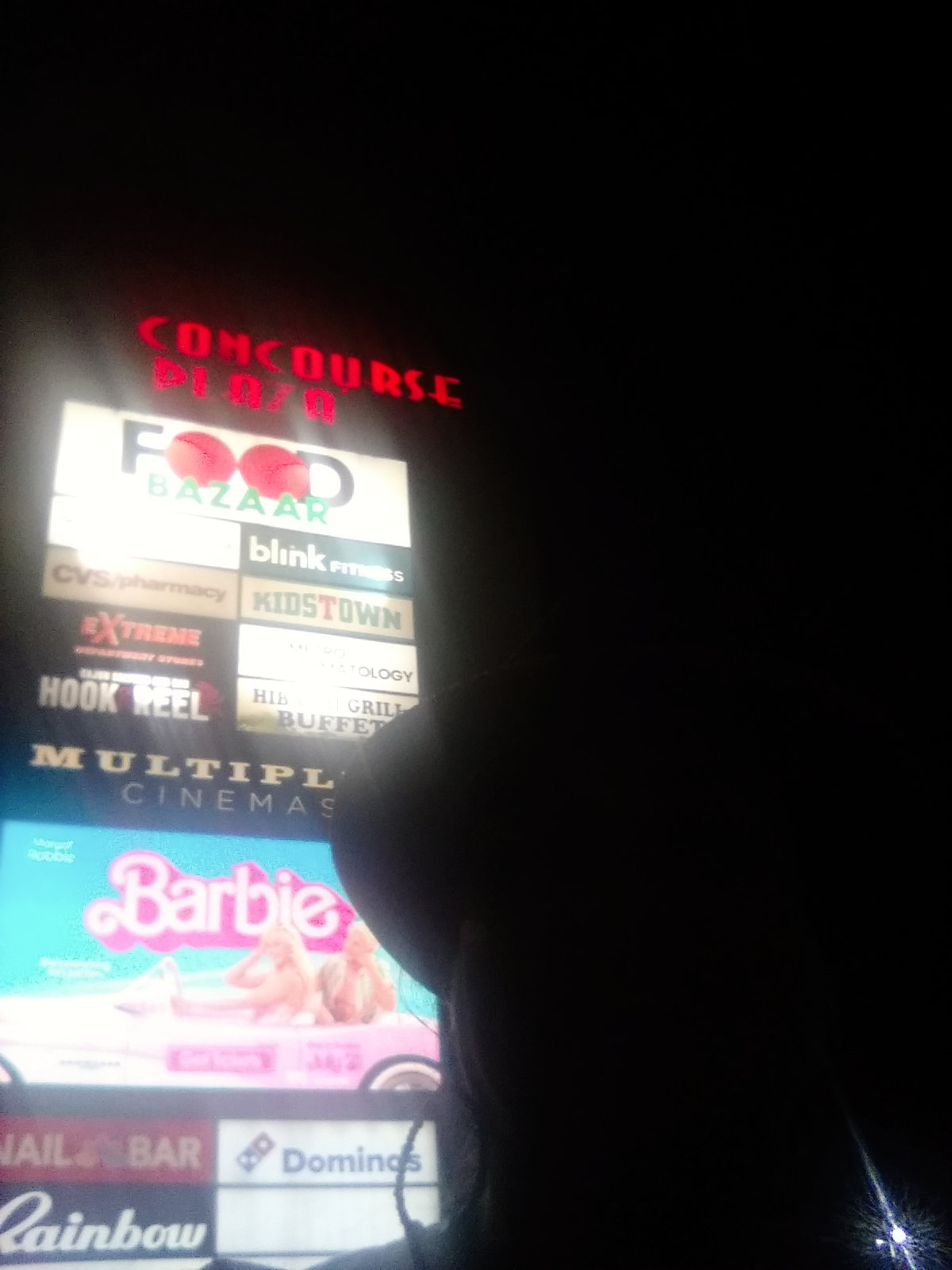The image features a bustling commercial plaza brimming with signage against a black background. At the top and right, the background appears pitch black, highlighting the vibrant signs adorned below. 

Starting from the top left corner, a white sign prominently reads "Food Bazaar." Adjacent to it, on the right, another white sign marks "Bling Fitness." To the further left, a sign announces "CVS Pharmacy." Following this pattern, "Kidstown" finds its place to the right. Moving downward, the next sign partially visible includes the word "Extreme," while to its right, a somewhat obscured sign ends with "ology." Further right, a sign for a grill buffet appears, followed by one for "Multiblood Cinemas." Below this cinema signage, there is a prominent poster for the movie "Barbie," featuring a blue background with two characters – a blonde woman and a blonde man – seated in a pink car.

Directly below the cinema sign, another sign reads "Domino's," showcasing the recognizable blue and red logo with blue text. Moving further right, a dark rectangle labeled with "Rainbow" in white text stands out. Beside it, an undecorated white rectangle perhaps awaits future signage.

The scene includes a silhouette of what appears to be a person standing in front of these signs, identifiable by the outline of their hair and hat, adding a dynamic element to the otherwise static yet vibrant backdrop.